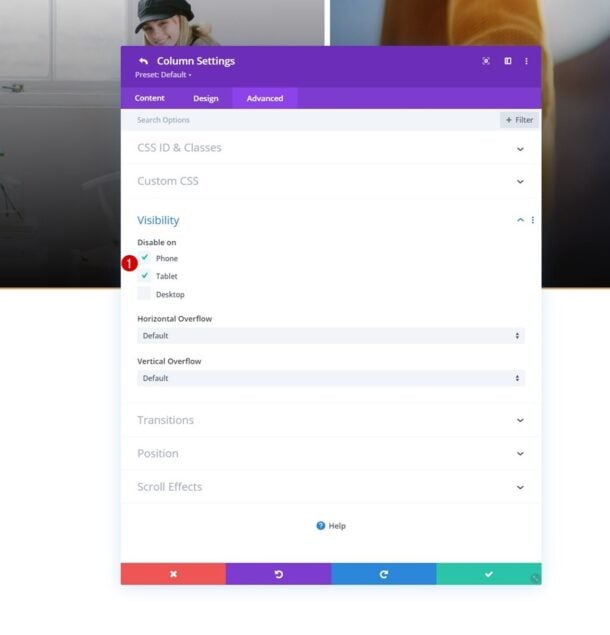The image consists of two side-by-side pictures, partially covered by a settings interface in the center. The left picture shows a scene with a white wall, a window, and a young woman wearing a black hat. The right picture is indistinct, featuring shades of brown and white with a black background.

In the center, the overlay interface displays a purple banner at the top labeled "Column Settings - Preset Default". Below this banner are three buttons: "Content", "Design", and "Advanced". Further down is a search bar with the text "CSS ID and Classes" and an adjacent drop-down arrow. Below the search bar, the text "Custom CSS" appears, also accompanied by a drop-down arrow. The section marked "Visibility" contains checkboxes for disabling the display on phones and tablets, both of which are checked and marked with green arrows. A red circular icon with the number "1" appears to the left of these checkboxes. The interface continues with options for "Horizontal Overflow" set to "Default", "Vertical Overflow" also set to "Default", and additional settings for "Transitions", "Position", and "Scroll Effects".